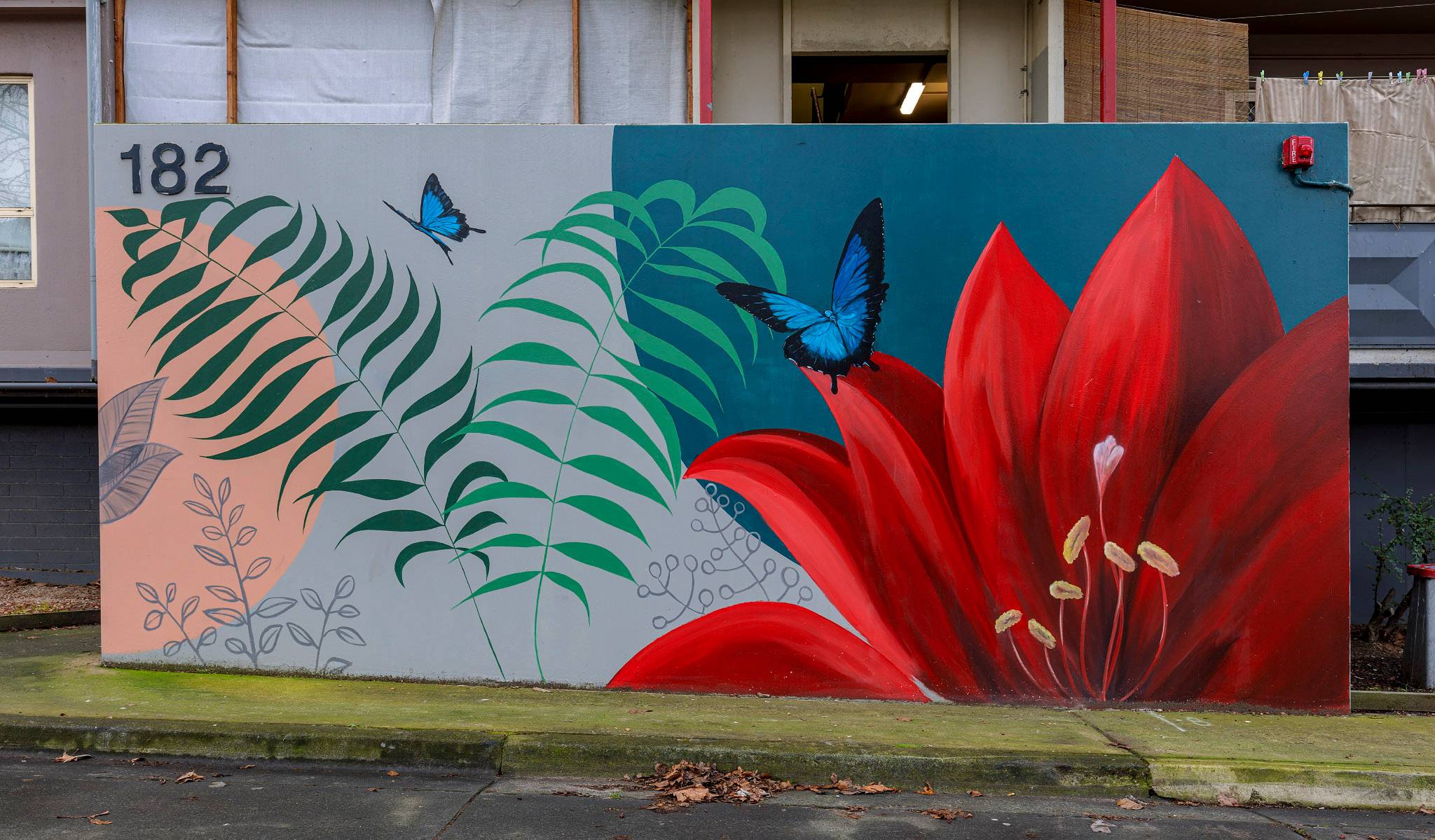A vivid rectangular painting hangs on what appears to be an outdoor sidewalk. Dominated by the number "182" in bold black letters on the top left corner against a gray background, the artwork features a captivating composition. The central focus is a vibrant, dramatic red flower with sharp, dahlia-like petals, outlined in black with lighter red highlights, creating a striking 3D effect. Adding to the scene's depth, a large blue butterfly with black-tipped wings rests on one of the flower's petals, while a smaller blue butterfly is also visible. The painting is interspersed with various shades of green leaves, with one stem dark green and another in light green. Additional details include a peach-colored circle on the left and a blue background on the right side of the painting. The artwork, reminiscent in style of both a mural and graffiti, is painted directly onto a dirty, weathered sidewalk, making it an eye-catching yet serene piece in an urban setting.